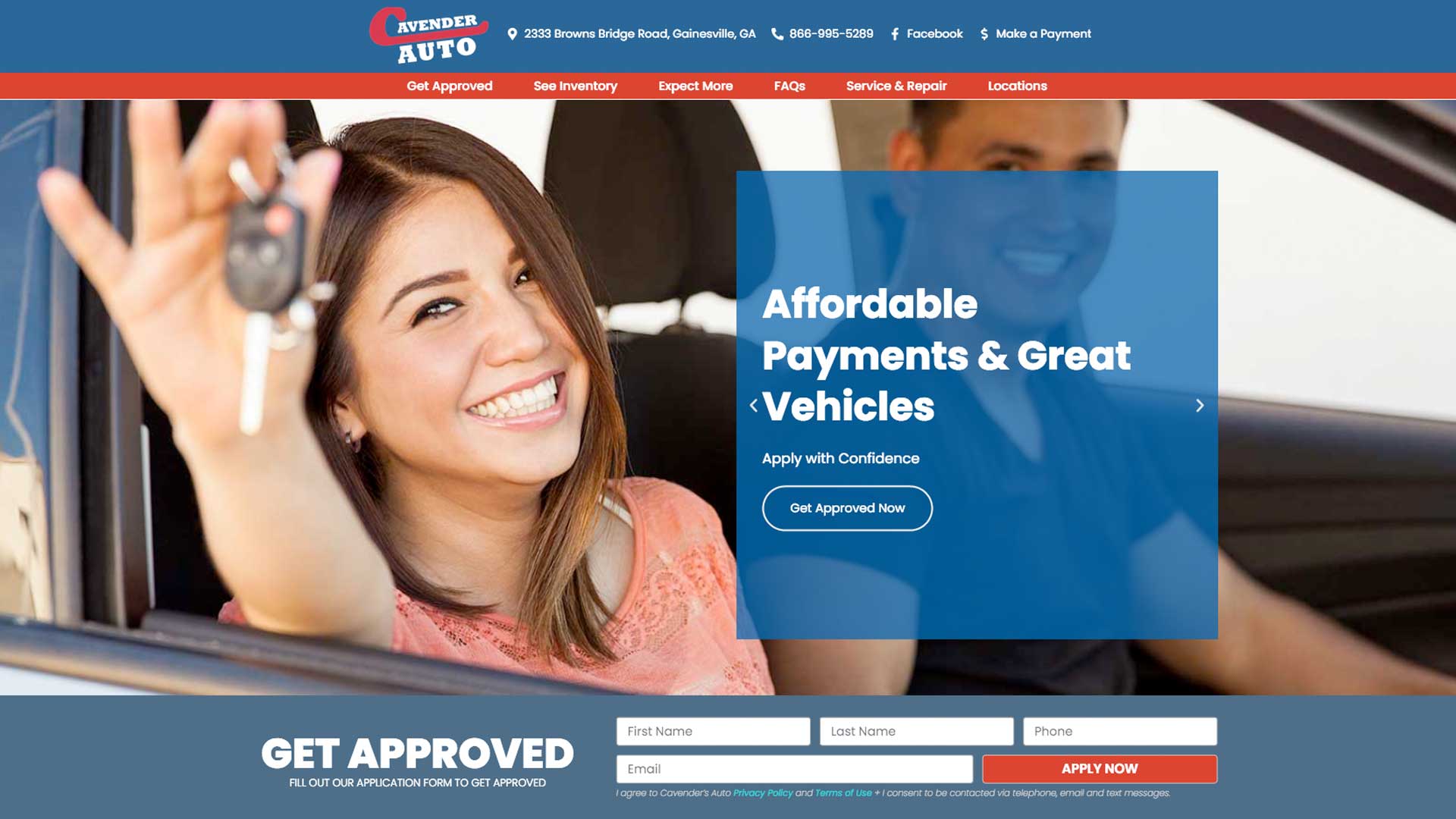**Detailed Descriptive Caption:**

The image depicts a webpage from "Avenger Auto," an automobile dealership. At the top, a blue banner with white text prominently displays the dealership's name, "Avenger Auto," flanked by a red emblem. Below the banner, the address "2333 Browns Bridge Road, Gainesville, Georgia," and phone number "866-995-5289" are clearly visible, alongside a Facebook icon and a "Make a Payment" option.

Directly beneath, another banner features a red strip with navigation options, including "Get Approved," "See Inventory," "Expect More," "FAQ," "Service and Repairs," and "Locations."

Below these banners, a large photograph captures a joyful moment between two young individuals inside a car. The woman in the passenger seat, with dark hair and light skin, wears a peach-colored shirt and is excitedly holding out a set of keys. The smiling man next to her also has dark hair and is dressed in a black shirt. 

A semi-transparent blue overlay is present in the image, partially obscuring the man's face. Over this overlay, white text reads: "Affordable Payments and Great Vehicles. Apply with Confidence. Get Approved Now."

At the bottom, a blue-gray strip invites viewers to "Get Approved" by filling out an application form, indicating fields for personal information below this line. This captures the welcoming and encouraging atmosphere of the dealership's website, emphasizing ease of approval and accessibility.